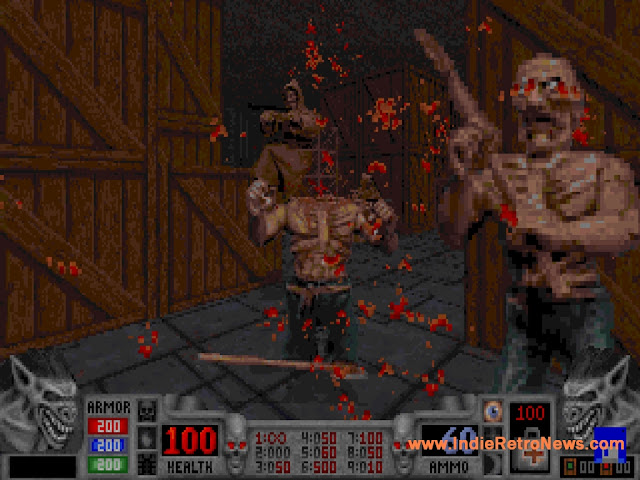This image depicts a scene from an old, pixelated 1990s to early 2000s video game, reminiscent of MS-DOS titles like "Quake." The game is a first-person shooter with a gray-hued interface. The bottom left corner features a detailed status HUD showcasing a gargoyle icon next to armor values displayed in red, blue, and green, each set at 200. There's also a health bar at 100%, along with additional information such as ammo count.

The scene itself is set in a warehouse with wooden boxes and gray tiles populating the background. The player character appears to be under attack from multiple monstrous entities resembling goblins, demons, or zombie-like creatures. One notable figure is a goblin-like creature with visible teeth. Blood splatters from the center of the screen imply a possible recent beheading, with an axe dropped nearby, heightening the grim atmosphere. Overall, the image captures a chaotic and bloody battle scene typical of classic horror-themed shooter games from that era.